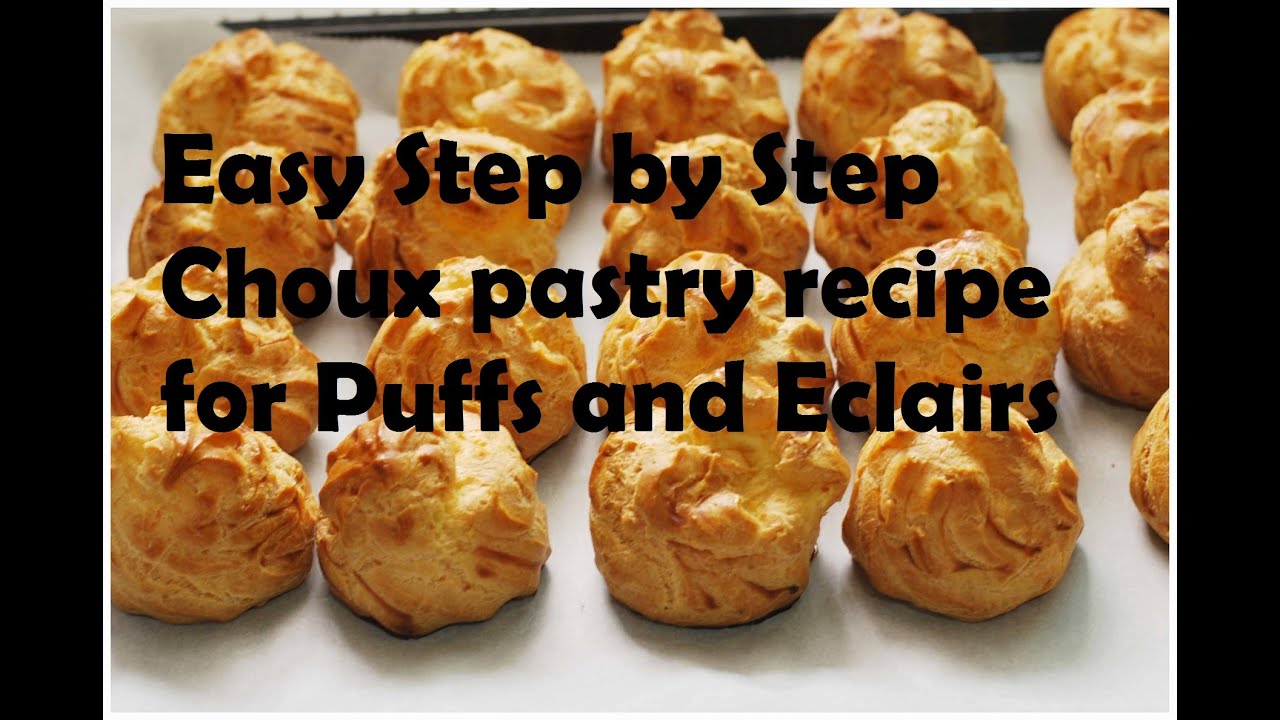The image depicts an arrangement of 20 golden-brown, round choux pastries, each with a swirled top, neatly placed in a 5x4 grid on a sheet of white parchment paper. The pastries are showcased on what appears to be a baking tray, flanked by black vertical bands on either side. Dominating the top part of the image, bold black text reads "Easy Step-by-Step Choux Pastry Recipes for Puffs and Eclairs." The visual emphasis is on the savory, golden hues of the pastries against the minimalistic black and white backdrop, drawing attention to the deliciously baked goods.